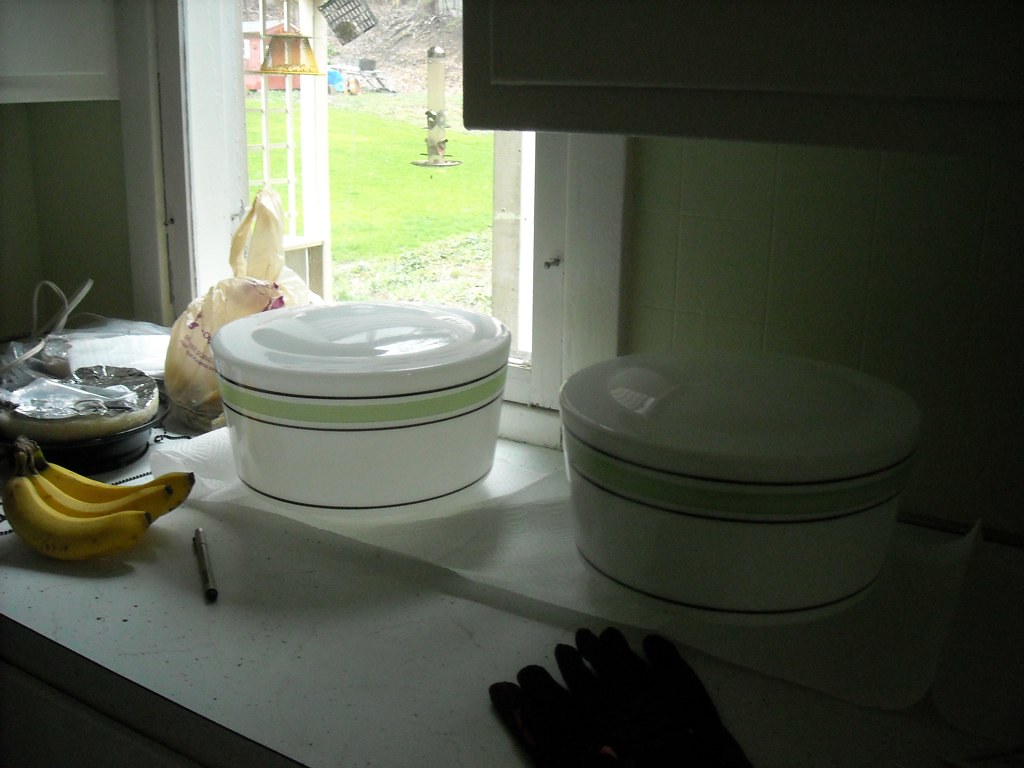In this dimly lit kitchen, illuminated by natural light streaming in from an open window to the left, various items are captured on the counter. The light from the window highlights a beige grocery plastic bag, knotted and possibly containing something, as well as a bunch of three bananas positioned at the edge of the counter. Next to the bananas lies a pen or mechanical pencil. A peculiar contraption, roughly the size of the banana bunch, also sits on the counter. It has a foil top and an uncertain purpose—potentially an ashtray or an incense holder.

Prominently featured are two large round Pyrex containers with decorative bands. The most visible container is white, adorned with a thick green band flanked by skinny white and dark blue bands, and comes with a lid. Its matching counterpart sits right beside it but is partially obscured by darkness. A pair of gloves is draped in front of this lesser-seen Pyrex. Through the open window, a bird feeder, a patch of green grass, and a red building are visible, adding a touch of the outdoors to this kitchen scene.